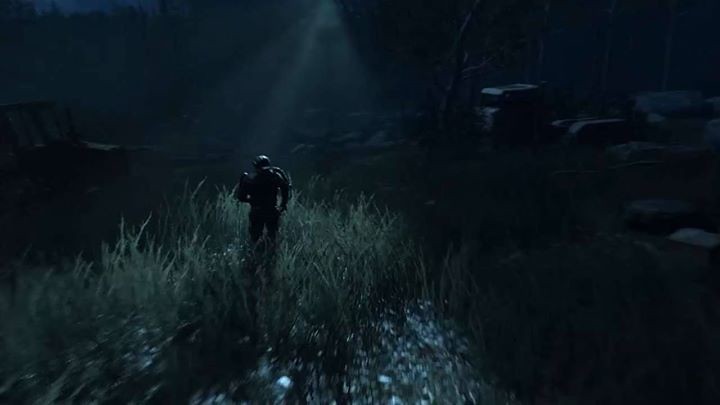The image, likely a still from a video game or a computer-generated scene, depicts a dark and desolate outdoor environment. Most of the picture is shrouded in black or very dark grey tones. A central light source, resembling faint moonlight, shines down towards the middle-left, casting dim illumination over the setting. Prominently featured is the silhouette of a humanoid figure, positioned slightly left of center and standing amongst tall grass. The figure's details are obscured by the darkness, but it appears to be wearing a science fiction-style outfit with a helmet and some kind of apparatus or tube extending from its back. There are hints of green on the figure, highlighted by the light. On the left side, faint outlines suggest the presence of a tractor or construction vehicle. The right side of the image fades into more obscurity, with some white, sharp-edged objects and the indistinct forms of possibly leafless trees, small buildings, or boulders. The overall mood is one of gloom and anticipation, accentuated by the shadowy, blurred background which hints at junked automobiles.